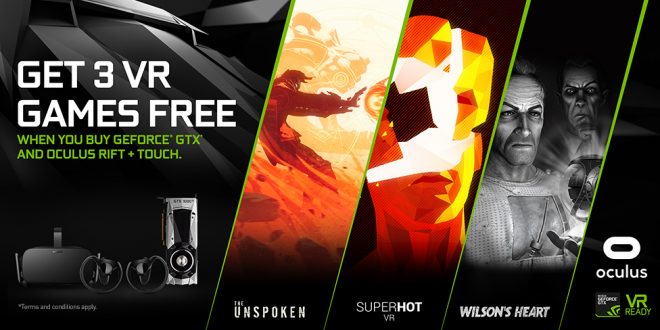The poster prominently announces a special promotion: "Get Three VR Games for Free When You Purchase GeForce GTX and Oculus Rift Plus Torch." The advertisement is visually striking, featuring bold text that highlights the offer. The background is likely designed to capture attention, possibly with graphics relating to virtual reality, such as futuristic imagery or game scenes. The message is repeated for emphasis, ensuring that viewers are clearly informed about the opportunity to receive three complimentary virtual reality games with the purchase of specified hardware. The logos of GeForce GTX and Oculus Rift are probably included, emphasizing the collaboration between these leading tech brands. This detailed promotional poster aims to entice gaming enthusiasts and tech-savvy consumers by offering an added value to their purchase.